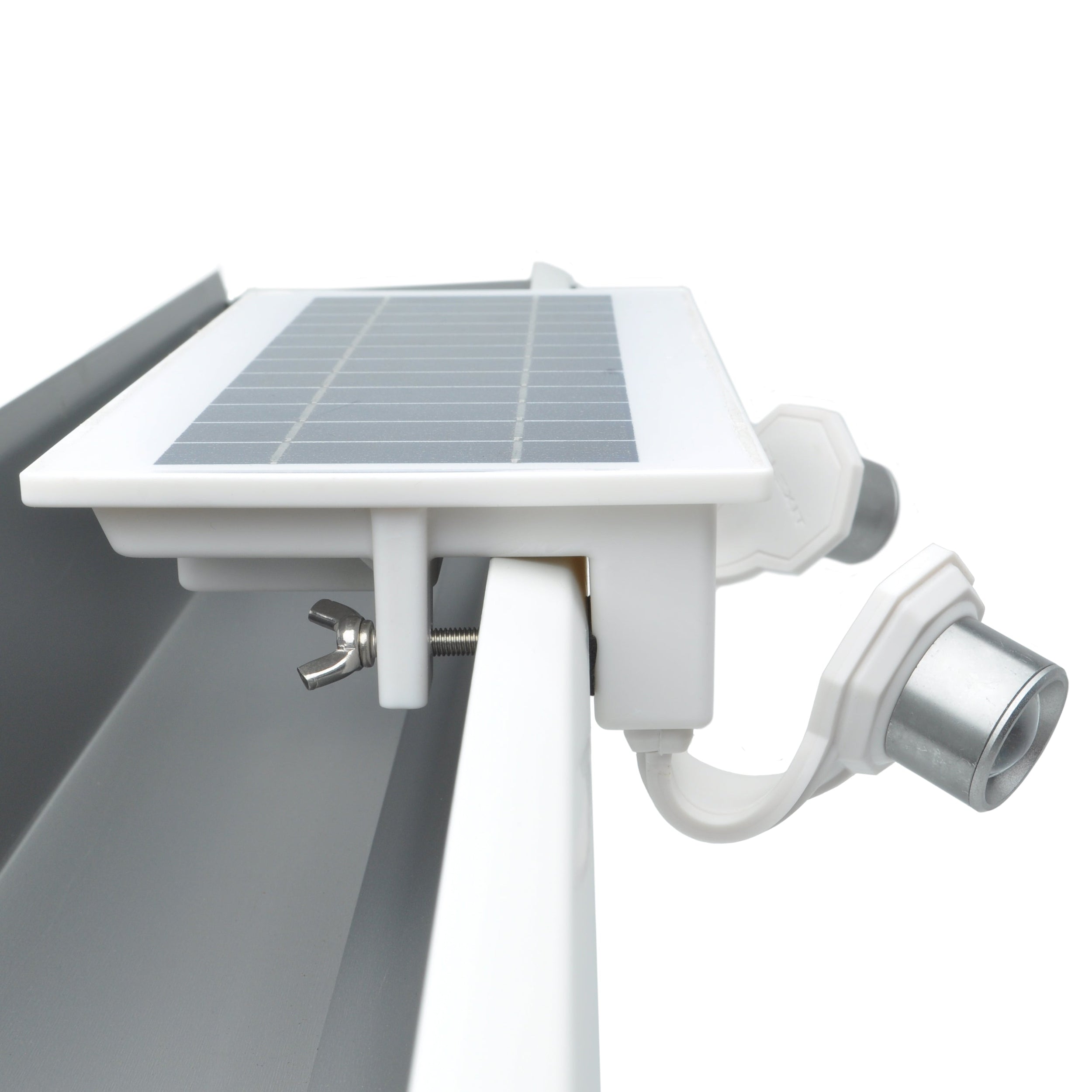The photograph depicts a highly detailed scene featuring a clamp apparatus attached to a white counter that appears to incorporate elements of a sink. The clamp itself is white with a silver screw, featuring a flat top area equipped with raised rubbery pieces to prevent slipping. On both the left and right sides of the clamp, there are silver lights facing the front, though they are not illuminated. The back handle of the clamp is also white. Below the clamp, a silver board is present, likely to catch sawdust or any falling debris. The background is entirely white, enhancing the visibility of the components in the image. Additionally, a silver cylinder, possibly a solar panel-like structure with a disc shape, extends from the white plastic part of the setup. This silver cylinder seems to connect the white shelving area to the gray interior, which could be part of a sink or another apparatus. The scene includes intricate details such as the silver hooks on the right end of the panel, adding complexity to the overall structure.